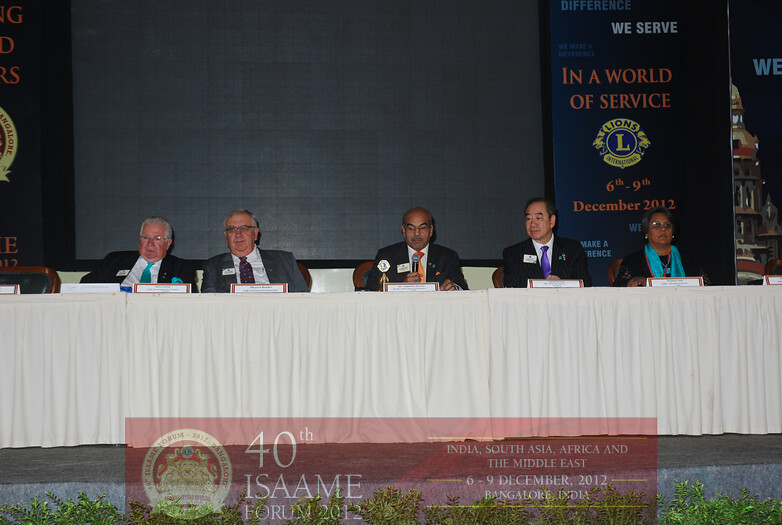Seated behind a long table draped with a white cloth, five distinguished individuals participate in a conference. The table, adorned with rectangular name cards, features attendees from various backgrounds. On the far left, an older man with gray hair, glasses, a dark gray jacket, white shirt, and a teal tie leans back in his chair. Adjacent to him is another gray-haired man in a gray suit with a dark purple tie, also wearing glasses. Centered at the table is a dark-skinned man with prominent brown eyebrows and a bald head, dressed in a black jacket, white shirt, and orange tie. He speaks into a microphone held before him. To his left is an East Asian man with short, graying black hair, who sports a black jacket, white shirt, and pink tie. On the far right sits a woman with dark brown skin, short gray hair, glasses, and a teal scarf around her neck, paired with a black shirt.

Behind them, a large banner with a dark blue background prominently displays the text, "We Serve in a World of Service," with a lion emblem and the dates "6/9 December 2012." Below, another semi-transparent banner reads, "40th Assam A Forum 2012, India, South Asia, Africa, and the Middle East, 6/9 December 2012, Bangalore, India." An empty chair with wooden edges and a blue cushion on the back sits at the left end of the table, emphasizing the organized yet formal setting of this gathering.